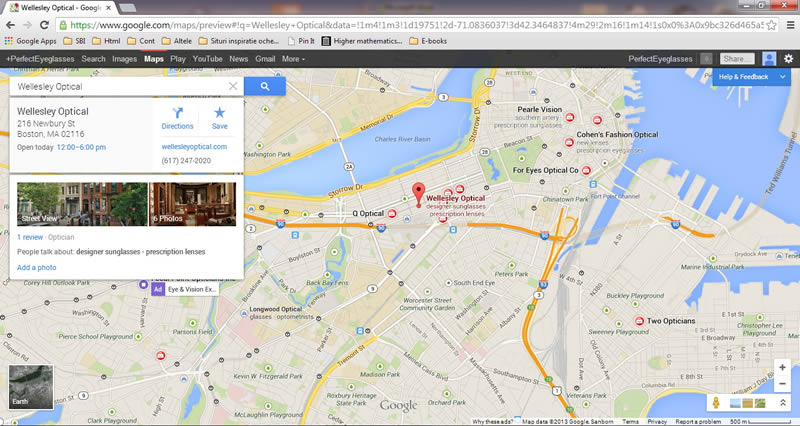The image is a horizontally rectangular screenshot of a computer screen featuring a search for Wellesley Optical on Google. At the top left, the browser tab displays the title "Wellesley Optical - Google." Directly beneath the tab is the web address bar. Below the address bar, there's a small toolbar with various links and icons labeled, though some are difficult to read due to their small size, including "Google Apps," "SBI," "HTML," and "E-Books."

Further down, there's a black navigation banner featuring categories such as "All," "Images," "Maps" (highlighted in bold), "Play," "YouTube," "News," "Gmail," and "More." 

Occupying the main portion of the screen is a map of Boston, Massachusetts, with a central marker pointing to the location of Wellesley Optical. In the upper left corner of the map, there's an overlay window presenting detailed information about the store. This information includes the store's address at "2016 Newbury Street, Boston, Massachusetts, 02116," and its operating hours for the day, which are "12-6." To the right of this information are two buttons for "Directions" and "Save." The window also lists the store's phone number and website.